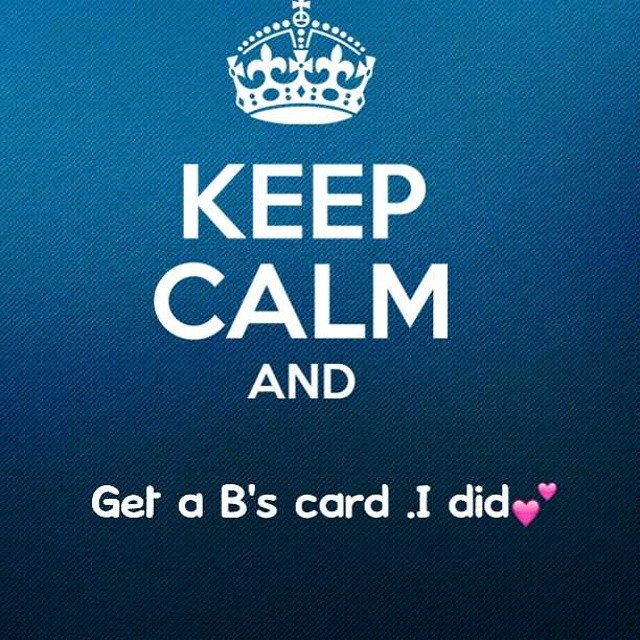The image features a textured dark blue background, reminiscent of denim, which fades in an ombre style from a lighter shade at the top to a darker one at the bottom. Centered at the top is an ornate white crown. Below the crown, in large white block capital letters, is the phrase "KEEP CALM," followed by a smaller, centered "AND" in the same font and color. At the bottom, in white Comic Sans font, it reads "get a bee's card. I did," accompanied by two pink heart emojis. The overall design mimics the iconic World War II "Keep Calm and Carry On" poster, blending classic elements with a modern twist.